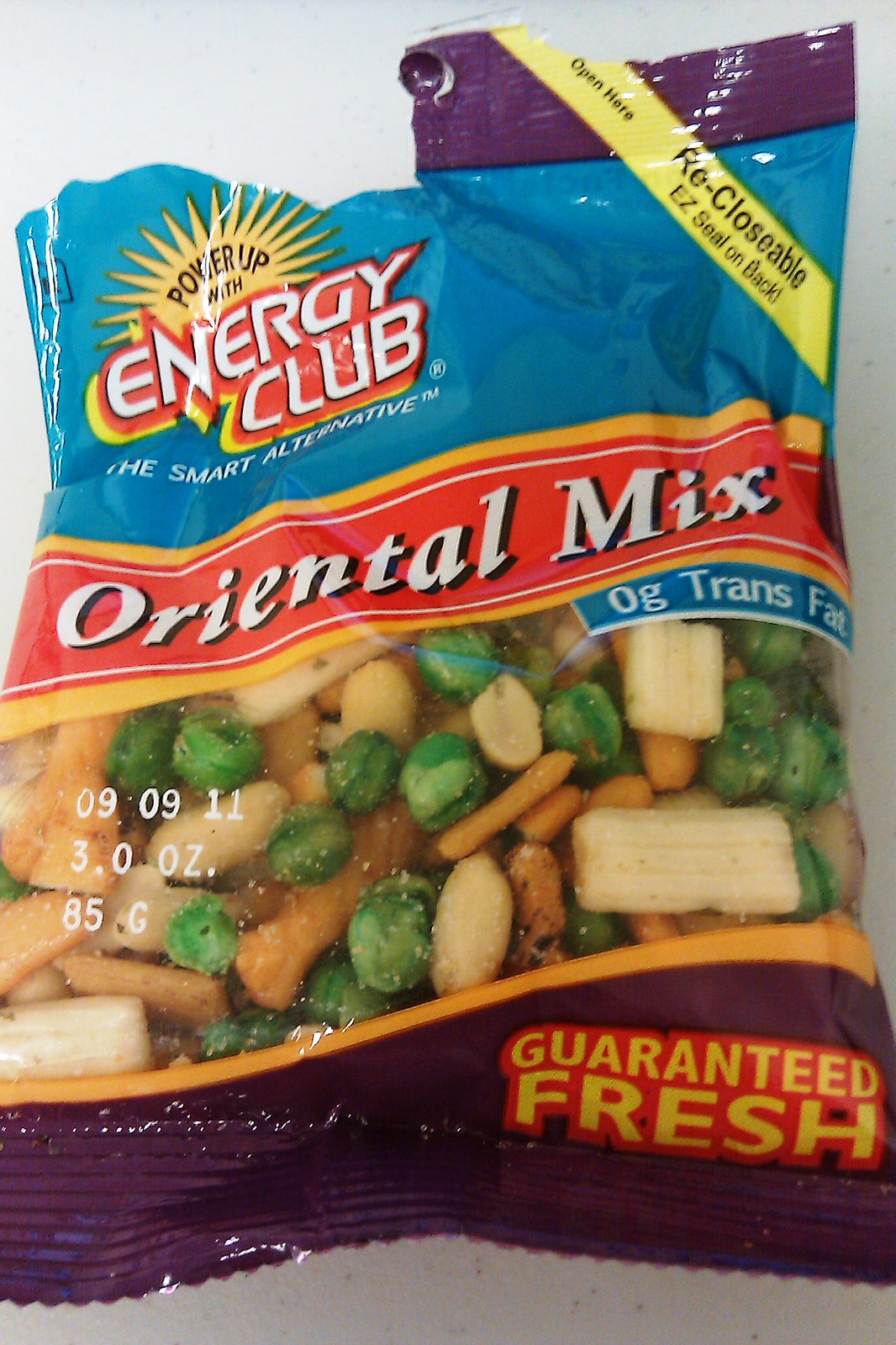This detailed close-up photo features a bag of dried snack vegetables, prominently labeled "Oriental Mix." The top of the bag has partially torn sections, which reveal several layers of design elements: an upper section in light blue with the text "Power Up with Energy Club, the Smart Alternative," a middle orange banner that states "Oriental Mix, 0% Trans Fat," and a yellow strip in the upper right corner that reads "Open Here, Reclosable, Easy Seal on Back." Below the orange banner is a clear window through which you can see a variety of dried vegetables, including baby carrots, bamboo shoots, green peas, and some round yellow and green vegetables. The bottom of the bag features a dark purple area with "Guaranteed Fresh" written in yellow outlined in red.